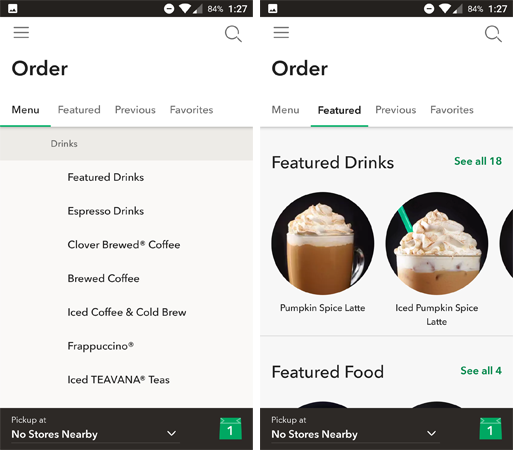This photograph showcases the interface of a food ordering mobile application, split into two distinctive sections side by side. 

In the left section, a white background dominates the top part with the word "Order" prominently displayed in black text. Below, various categories are listed, starting with "Menu" which is highlighted with a green underline. Following the menu, the "Drinks" category is selected, presenting options such as "Featured Drinks," "Espresso Drinks," "Clover Brewed Coffee," "Iced Coffee and Cold Brew," "Frappuccino," and "Iced Teavana Teas." Towards the bottom, there is a black rectangular box with white text indicating "Pick Up At," but currently, it displays "No Stores Nearby." Additionally, there is a number "1" in white text enclosed within a green circle located on the left side of the section.

The right section mirrors the left in its white background and top header featuring the word "Order." Here, "Featured" is highlighted with a green underline. This section includes a visual display of featured products starting with a heading "Featured Drinks" followed by an option to see all 18 items. Below this, round image thumbnails on a black background depict a "Pumpkin Spice Latte" and an "Iced Pumpkin Spice Latte." The lattes are richly caramel-colored, served in clear glasses, topped with foam or whipped cream, with the iced variant featuring a green straw. Beneath the drinks section, "Featured Food" is mentioned with an option to see all four items in green text. This section, too, includes the black rectangular box stating "Pick Up At" and "No Stores Nearby," along with a number "1" in white text encased in a green square.

Together, these sections provide a detailed view of the user's menu navigation and current selection status within the mobile application.